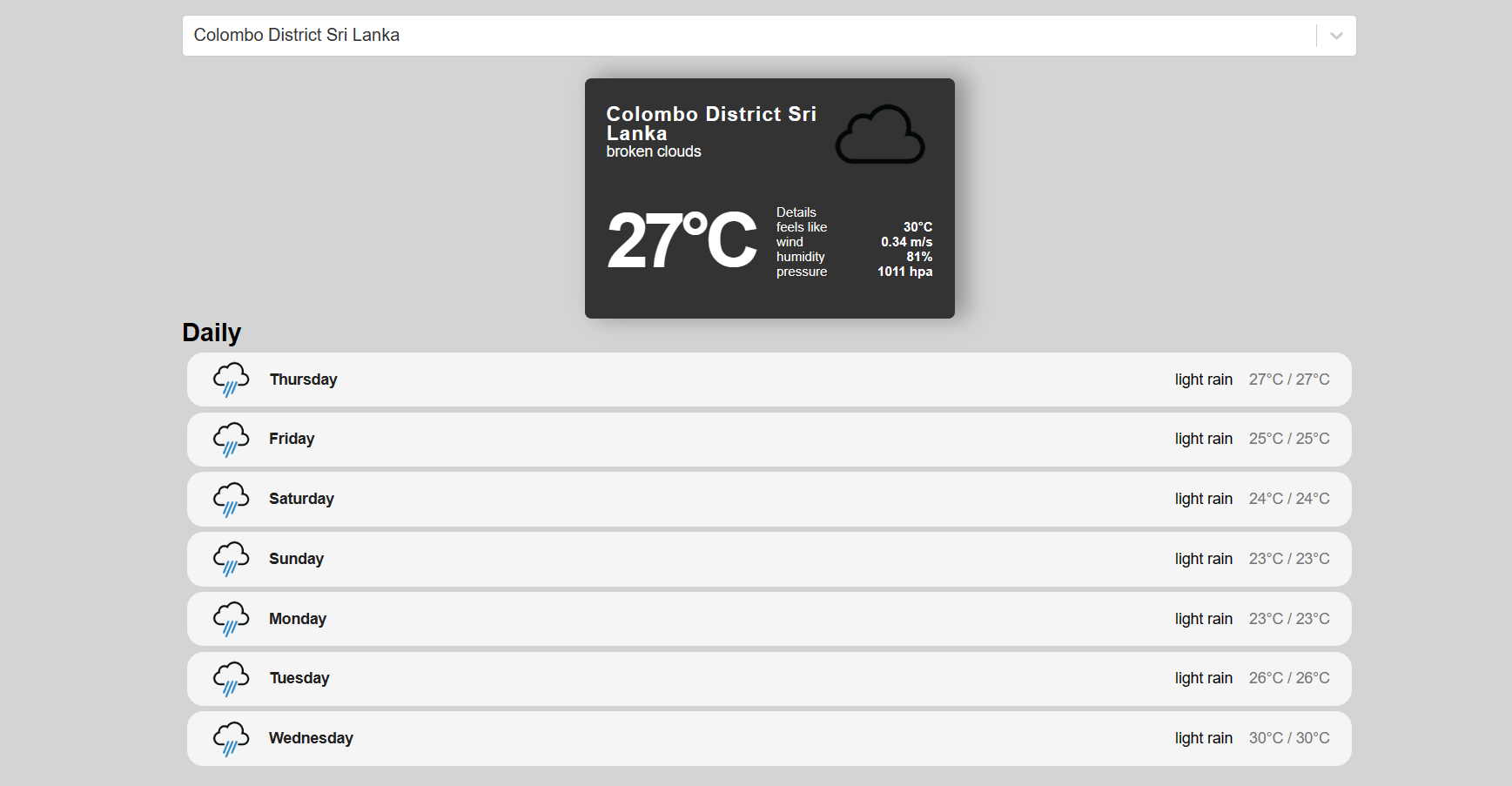The image is a horizontally rectangular screenshot with a predominantly grey background, displaying detailed weather information for Colombo District, Sri Lanka. At the top center, there is a white dropdown field on the right side labeled "Colombo District, Sri Lanka."

Below this, in the central portion of the image, a black square contains basic weather information, which reads:
- Colombo District, Sri Lanka
- Broken clouds
- 27 degrees Celsius
- Feels like 30 degrees Celsius
- Wind: 0.34 km/h
- Humidity: 81%
- Pressure: 1011 HPA

Underneath this section, horizontal bars represent the weather forecast for the upcoming days of the week. Just above these bars on the left side, the label "Daily" is displayed. Each day of the week is listed vertically with corresponding weather predictions:
- Thursday: Light rain
- Friday: Light rain
- Saturday: Light rain
- Sunday: Light rain
- Monday: Light rain
- Tuesday: Light rain
- Wednesday: Light rain 

Overall, the forecast indicates a consistent trend of light rain throughout the week.